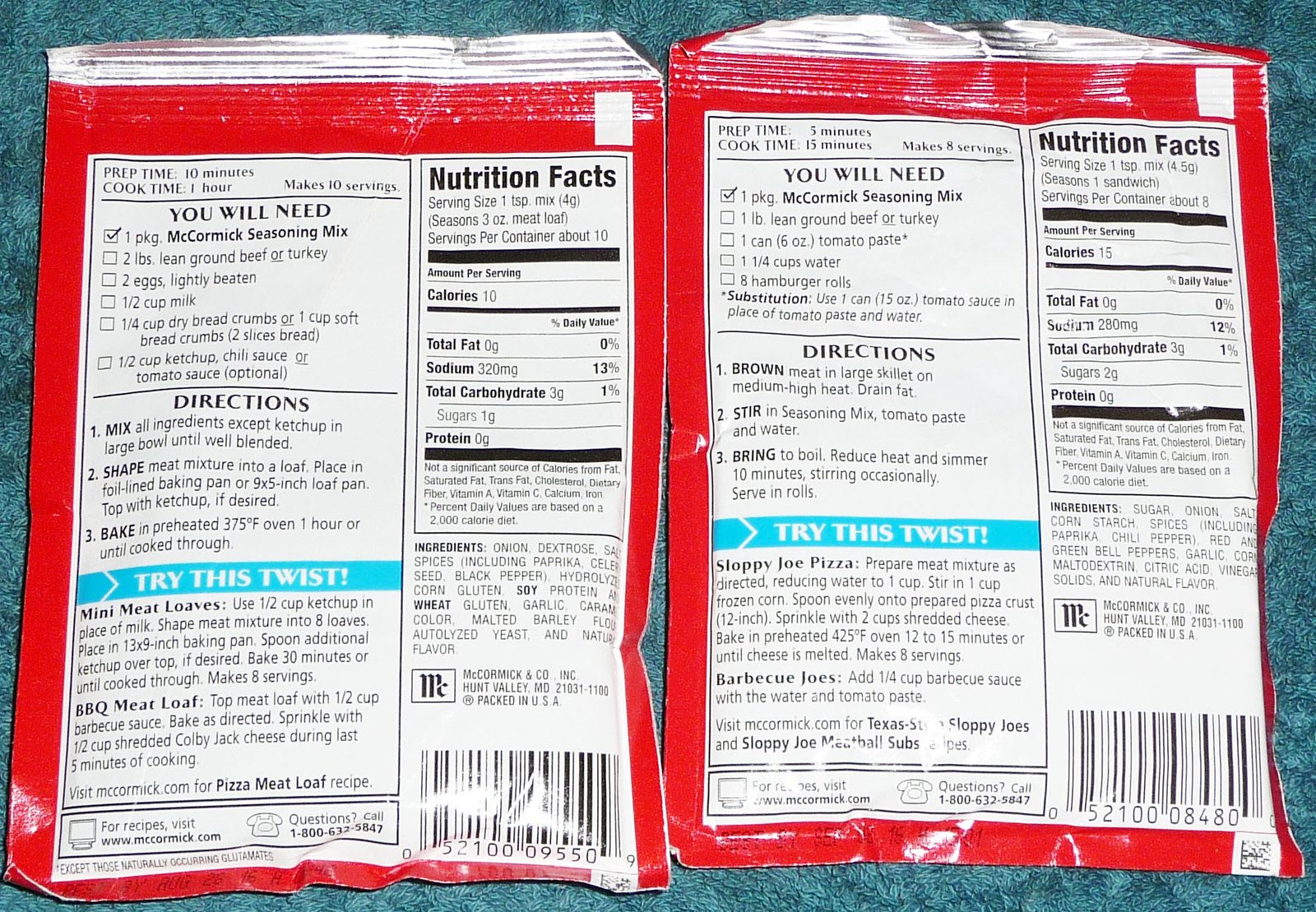The image features two McCormick & Co. seasoning mix packets, both prominently displayed against a teal-colored, carpet-like background. Each packet is red with a white interior section, accented by a silver strip along the top. 

**Left Packet:**
- **Design:** Red border with a white interior and a silver strip on top. 
- **Details:** It states a preparation time of 10 minutes, a cook time of 1 hour, and yields 10 servings.
- **Nutritional Information:** 10 calories, 0g fat, 320mg sodium, 3g carbohydrates, 1g sugar.
- **Additional Features:** Contains recipes for mini meatloaves and barbecue meatloaf. Text at the bottom encourages trying these twists.

**Right Packet:**
- **Design:** Similar to the left packet with a red border, white interior, and a silver top strip.
- **Details:** Indicates a preparation time of 5 minutes, a cook time of 15 minutes, and makes 8 servings.
- **Nutritional Information:** 15 calories, 280mg sodium, 3g carbohydrates, 0g sugar, and some protein content.
- **Additional Features:** Provides recipes for Sloppy Joe pizza and barbecue joes, also suggesting trying these twists.

The back of each packet showcases detailed nutritional information and recipe suggestions for dishes made with beef or turkey.